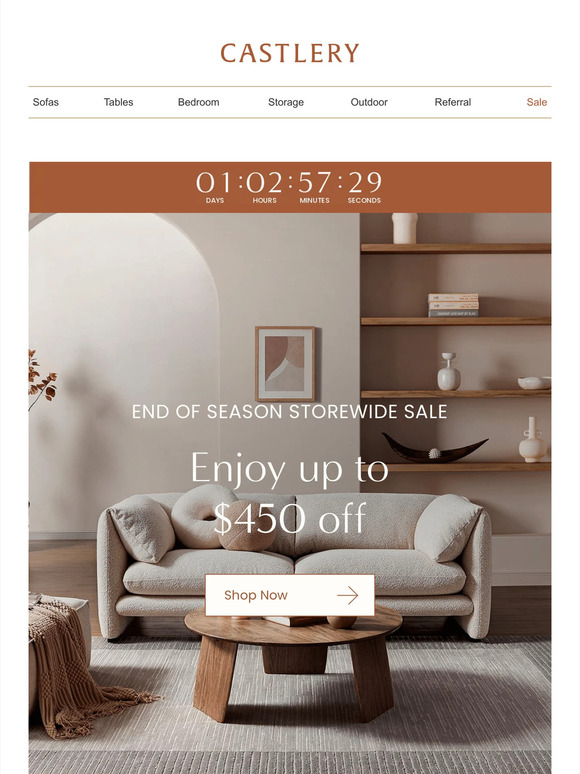This image appears to be an advertisement for an online store named "Casterly." The top of the image features the store's name in bold brown letters, centered on the page. Below the store's name, there's a navigation bar with clickable options such as "Sofas," "Tables," "Bedrooms," "Storage," "Outdoor," "Referral," and "Sale," with the word "Sale" highlighted in brown while the rest are in black.

At the very top, overlaid on the page, is a countdown clock displaying the remaining time for a sale, which is set to one day, two hours, 57 minutes, and 29 seconds. Below this timer, the image depicts a stylish and cozy living room setup. 

The living room features a two-tone gray rug that spans the floor area at the bottom of the image. A round wooden coffee table sits prominently on the rug, with a clickable white box above it that reads "Shop Now," accompanied by a right-pointing arrow.

Behind and above the coffee table stands a luxurious tan sofa adorned with matching tan pillows. Hovering above the sofa is text offering an attractive discount: "Enjoy up to $450 off." Further upwards, bold text announces the "End of Season Store-Wide Sale," drawing attention to the significant savings.

The background of the image showcases a wall painted in a warm tan color, decorated with a central geometric art piece in shades of brown, tan, and gray. To the right, a built-in wooden bookcase is filled with various books, vases, and a distinctive black bowl shaped like a canoe. On the far left edge of the image, a fragment of a plant and a chair draped with a blanket can be seen, adding to the cozy and inviting atmosphere of the scene.